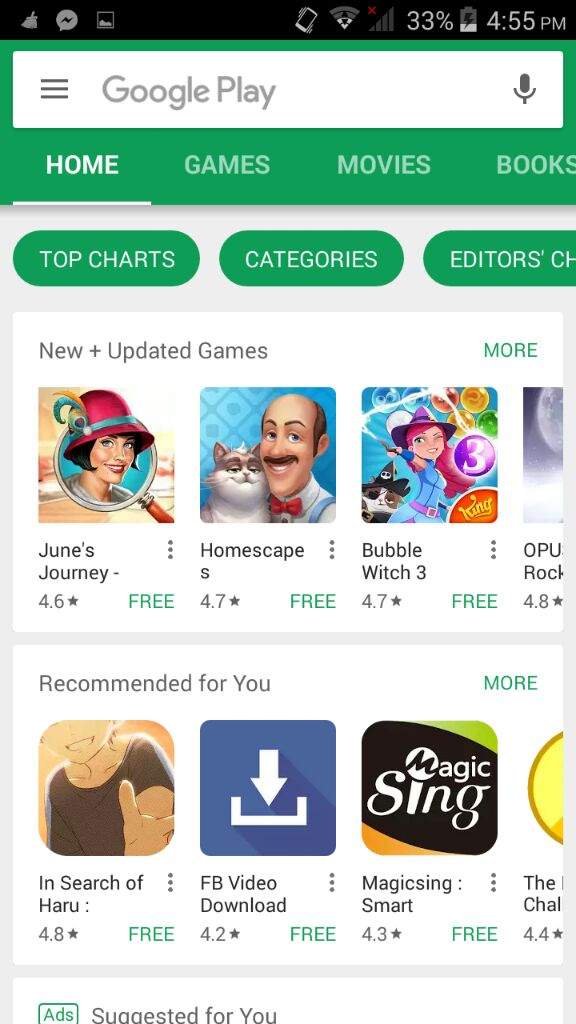The image depicts a detailed screenshot of the Google Play Store interface. The top of the screen features a blue background with a right-pointing arrow and a circular icon containing a black squiggly line and a small gray element, flanked by indicators showing "33%" battery and the time "4:55 PM."

Below this header, a large white search box is centered, containing three horizontal lines (menu icon), the text "Google Play," and a microphone icon. The interface then shifts to a green section highlighting various tabs such as "Home," "Games," "Movies," and "Books," with "Home" being underlined, indicating it's the currently active tab.

Beneath these tabs, another blue background section displays three prominent green buttons labeled "Top charts," "Categories," and "Editor's choice."

The main content area features a white box titled "New & Updated Games." This section showcases a list of games accompanied by their ratings and pricing information: 
1. "June's Journey" rated 4.6 stars, free.
2. "Homescape" rated 4.7 stars, free.
3. "Bubble Witch 3" rated 4.7 stars, free.
The fourth game in this list is partially cut off.

Following another blue section, there's a second white box labeled "Recommended for You," presenting another series of apps:
1. "In Search of Haru" rated 4.8 stars, free.
2. "Facebook Video Download" rated 4.2 stars, free.
3. "Magic Sing Smart" rated 4.3 stars, free.
Again, the fourth app in this list is cut off.

Further down, another white box with the label "Ads" in green and partially encased in a blue outline shows the "Suggested for You" section.